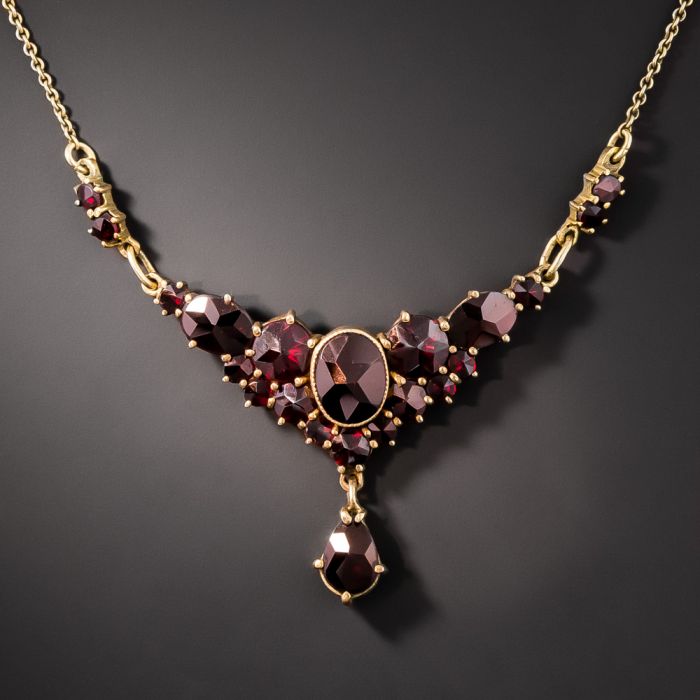This large-square image showcases an exceptionally elegant and sophisticated necklace, intricately designed in gold. The necklace features a delicate chain with small links that originate from the upper left and upper right corners of the image. These small links transition into larger chain links adorned with deep, rich burgundy-colored gems that resemble rubies or amethysts.

As the necklace draws towards the center, it boasts a prominent pendant area. This centerpiece is a striking arrangement of larger gems matching those on the chain. It includes a circular gemstone with a thin gold rim, accompanied by a more pronounced teardrop-shaped gemstone that dangles elegantly beneath it, framed by a gold ring and three small gold notches.

The background of the image is a solid dark gray, nearly black in the lower left and right corners, which starkly contrasts and highlights the brilliant, dark red stones and gold elements of the necklace. The overall design forms a heart-like shape and exudes an impression of high value and opulence, suggesting it’s a piece that would be worn by someone of distinguished taste.